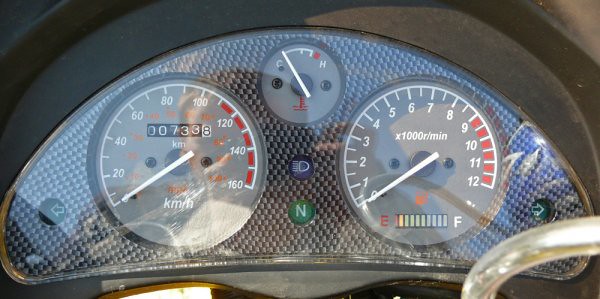The image depicts the control panel of a car, set against a dark gray background. The panel itself is black along the edges, with a glass-covered middle section that has a semi-circular shape, rounded at the ends. 

Prominently featured are three dials: two larger ones on the left and right, and a smaller one in the center at the top. The larger dial on the left is the speedometer, while the one on the right displays the engine's RPM (revolutions per minute). The smaller, central dial at the top indicates the fuel level.

Additionally, there is a small blue square with a semi-circle and radiating lines, alongside a green button with a white symbol in the center. Down in the corner on the right side, a semi-circular, almost clear plastic element extends outward, adding a subtle touch of functionality to the controls.